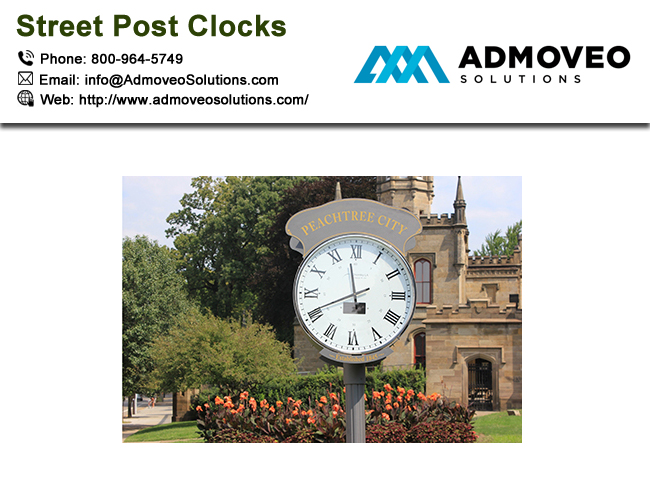This is a daytime color image featured in an online advertisement for street post clocks. The photograph prominently displays a standalone clock mounted on a street post at the center of the image, with the time displayed as 11:41 a.m. The clock bears the inscription "Peachtree City" at the top. Surrounding the base of the clock is a small flower garden with shrubs and a grassy area. To the left of the clock, there are trees, and to the right, there's a small stone building that bears a resemblance to a mini castle or church. Adjacent to this scene, on the left-hand side, is a sidewalk.

At the very top of the image, there is a letterhead and logo for AdMovio Solutions. The letterhead reads: "Street Post Clocks, Phone 800-964-5749, Email info@admoviosolutions.com and web http://www.admoviosolutions.com."